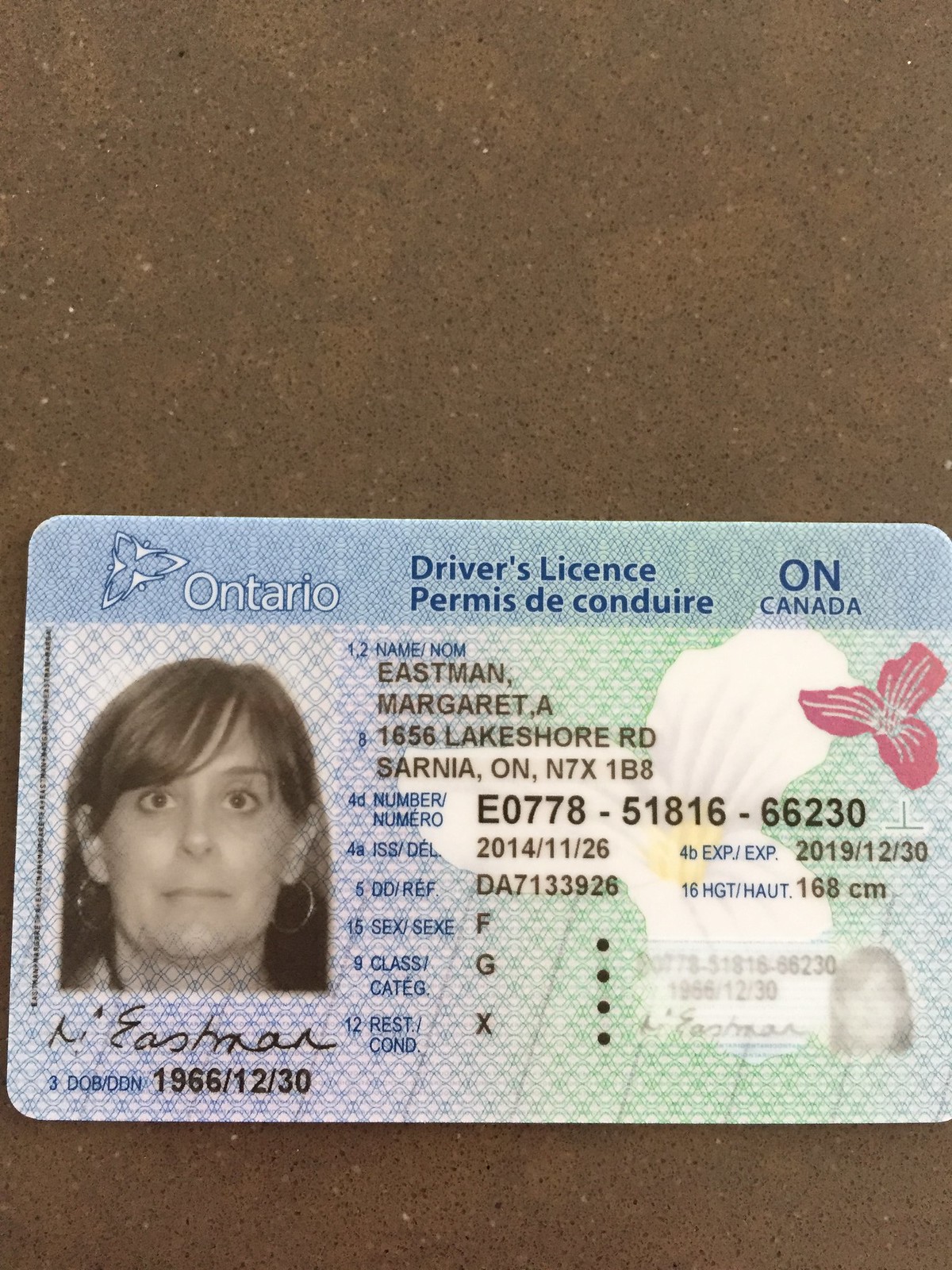The image depicts a single Ontario driver’s license laying flat on a brown stone or pegboard-like surface. The license belongs to a woman named Margaret A. Eastman, whose address is 1656 Lakeshore Road, Sarnia, Ontario, N7X 1B8. The ID features a detailed photograph of Margaret on the left side, where she appears with shoulder-length brown hair and circular silver earrings, staring intently at the camera. Beneath her photograph is her signature, accompanied by her date of birth: December 30, 1966. The license also displays various important details such as her license number: E0778-51816-66230, issue date: November 26, 2014, and expiration date: December 30, 2019. Additional information includes her height: 168 centimeters, sex: Female, license class: G, and a reference number: DA7133928. The driver’s license is offset slightly towards the bottom center of the image, which is taken indoors, lending a homey background color palette of browns, light blues, greens, pinks, whites, and yellows.